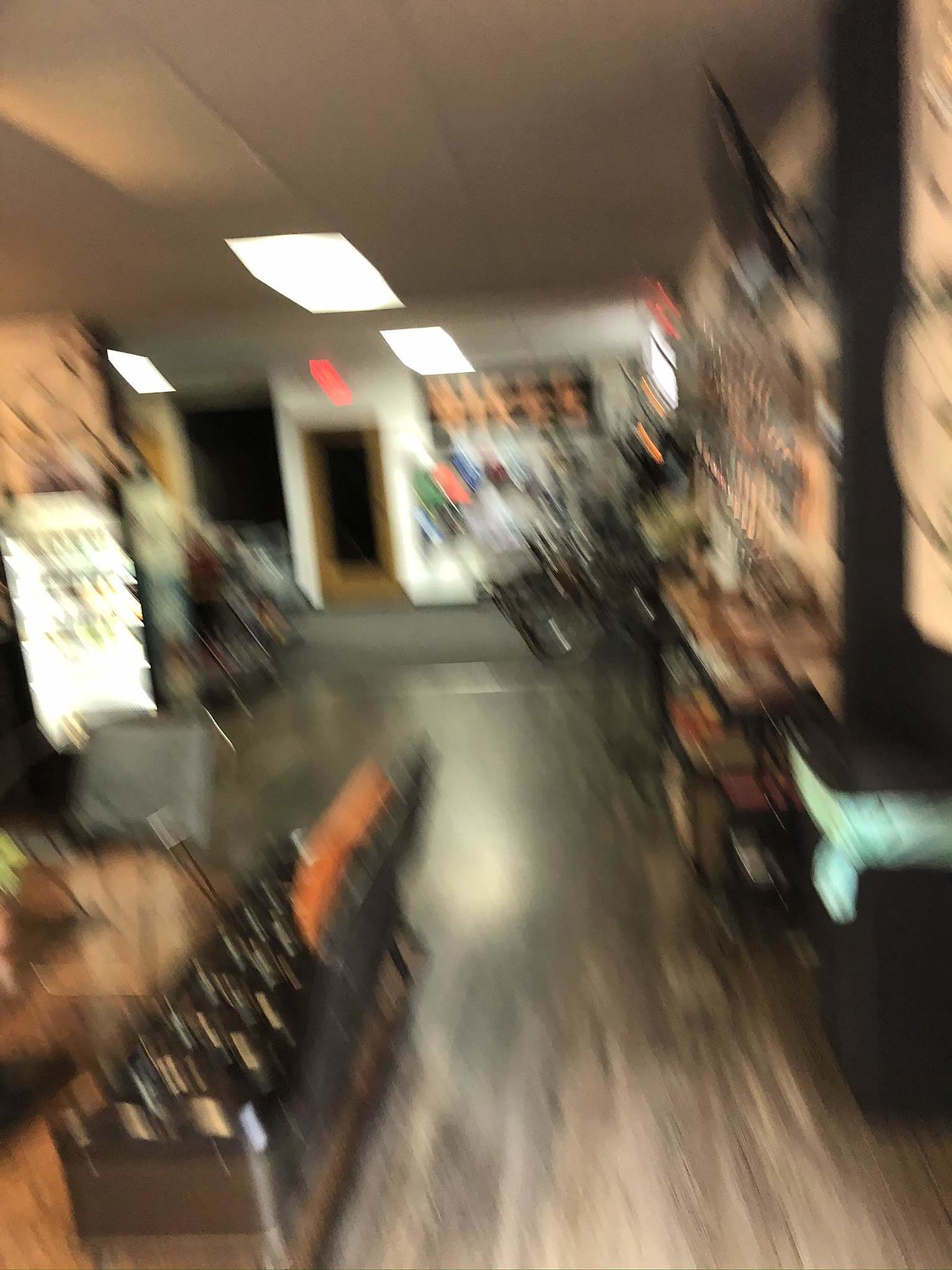This image, which is vertically oriented and notably blurry, captures the interior of what appears to be a wine store. The scene unfolds down a store aisle, showcasing a glossy wood grain floor that could either be real wood or laminate. A blurry figure can be seen walking towards the viewer in the background, adding a dynamic element to the otherwise still environment.

On the bottom left, a tall, thin box extends upwards, seemingly housing wine bottles. Along the right-hand side, tall shelves stretch all the way to the ceiling, likely lined with various bottles and merchandise. In the background, a door is visible, marked by an exit sign above it. The ceiling features acoustical panels interspersed with recessed UV lighting rectangles, illuminating the space softly yet distinctly.

Additionally, a display case on the left side of the aisle stands out as a brighter element, possibly highlighting special or premium products. Despite the overall blurriness of the image, these details contribute to an impression of a cozy yet sophisticated retail atmosphere.